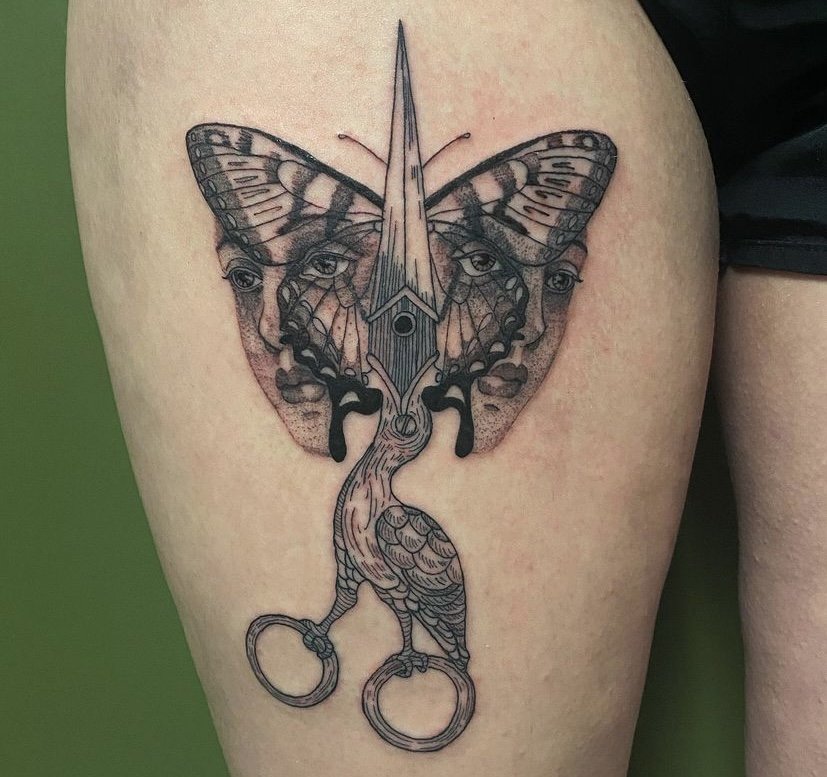This close-up photograph captures a detailed tattoo on the front of a woman's thigh, extending from near her hip down to the top of her knee. The tattoo features a central pair of scissors designed to resemble a bird, with the bird's body forming the handles of the scissors. The bird's head points upwards, with the scissors' blade extending from its beak towards the sky. Intricately woven into this design is a butterfly, whose wings are adorned with the solemn profiles of two women's faces, each facing outward. Adding to the complexity, a small house or birdhouse appears in the middle where the scissor blades meet. The tattoo is primarily rendered in intricate black line work, with touches of red shading. The background of the photograph shows a light green color, enhancing the contrast of the black ink. The woman, who is Caucasian and wearing shorts, stands against the green backdrop, highlighting the elaborate and symbolic art on her skin.